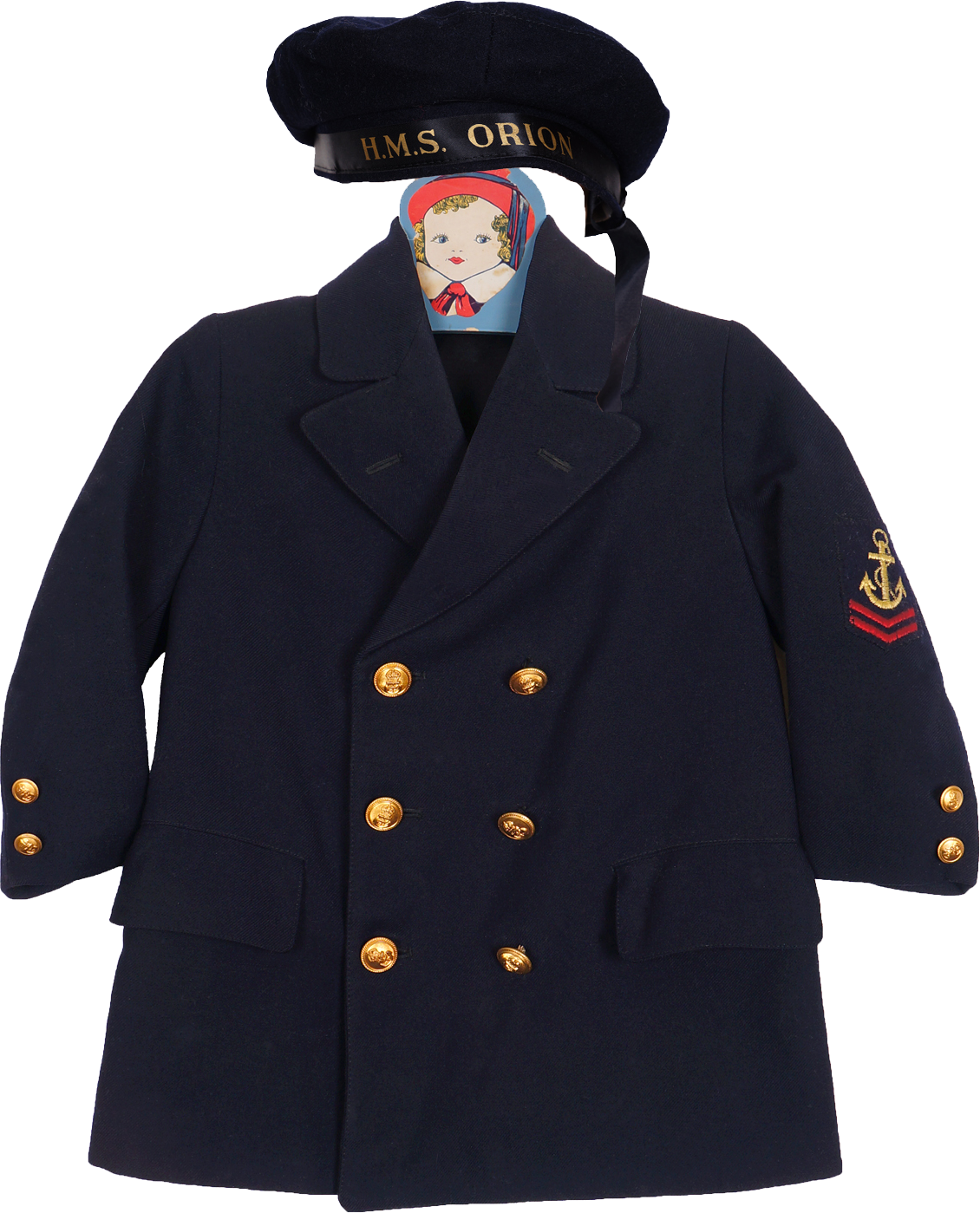The image is a rectangular photograph with a white background, featuring a dark navy blue sailor's uniform designed for a child. The costume appears to be floating in an empty white void due to image editing. The uniform includes a double-breasted wool coat adorned with a series of six metallic gold buttons on the front and two gold buttons on each cuff. The front of the coat also features two pockets. On the right sleeve, there is a blue patch with a golden anchor and two red chevrons beneath it. Above the coat, a small navy blue cap with a blue tassel on the right side and gold text around the band reading "HMS Orion" is displayed. The coat hanger is a picture of a baby wearing a red cap and a white shirt.